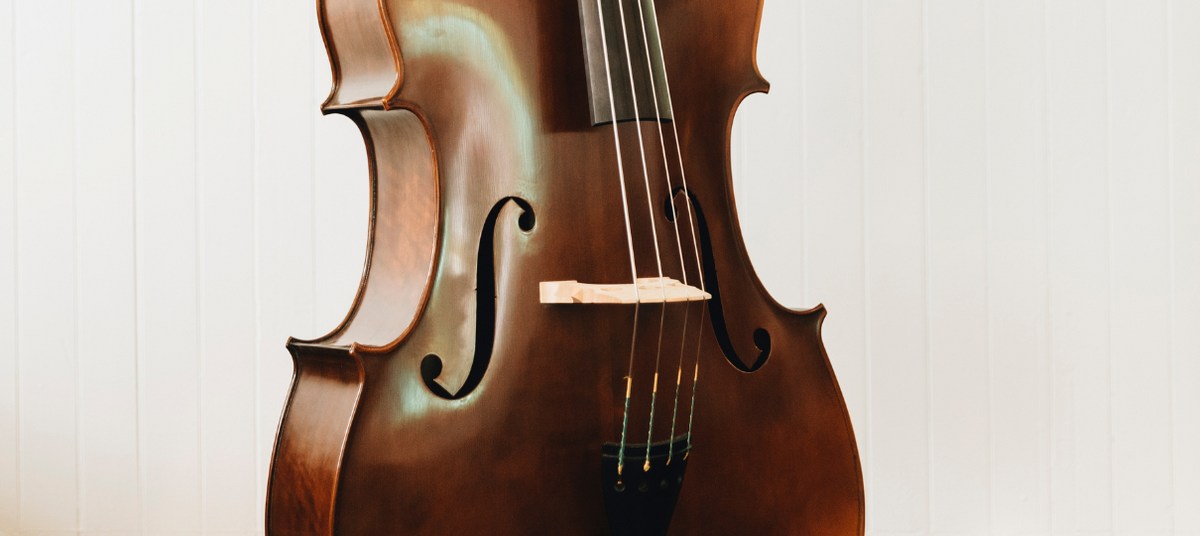The photograph captures a close-up of a brown, shiny violin placed against a white wooden background. The focus is on the body of the instrument, showcasing its dark wooden finish and the intricate S-shaped sound holes, also known as f-holes. The highly polished surface of the violin reflects light beautifully. The image highlights the four silver strings, stretched taut across the body, leading to a black tuning apparatus at the bottom. Additionally, there is a white guiding string to help align the main strings properly. Notably, the photograph excludes the neck and the very bottom of the violin, emphasizing the central portion of this elegant string instrument.